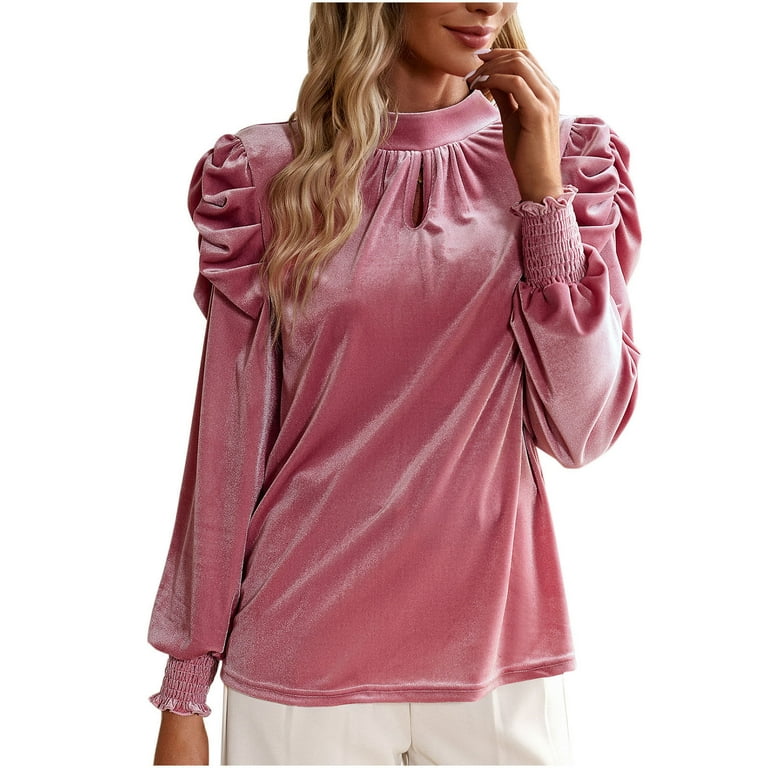This product image captures a woman wearing a striking pink tunic blouse with a velvety, satiny finish that shimmers under the light. The focus is on the flowing, soft fabric of the blouse, which drapes elegantly over her torso. The blouse features ruffled details at the shoulders and a teardrop-shaped neckline that adds a delicate touch near her throat. The long sleeves are ruched, with the fabric cinching around the wrists in a stretchy, tight design, complete with small ruffles at the cuffs. The woman's white complexion and long, wavy blonde hair frame the blouse, although her face is partially obscured, with the image cutting off just below her nose. Her left hand is delicately raised near her lips, and she sports white nail polish and pink lipstick that complements the blouse. The background is a clean, white backdrop, further emphasizing the soft, luxurious appearance of the blouse. She is also wearing white shorts, but they are not the focal point. The overall presentation suggests a formal yet comfortable appeal, with a visually captivating contrast between the blouse’s rich texture and the simplicity of the setting.